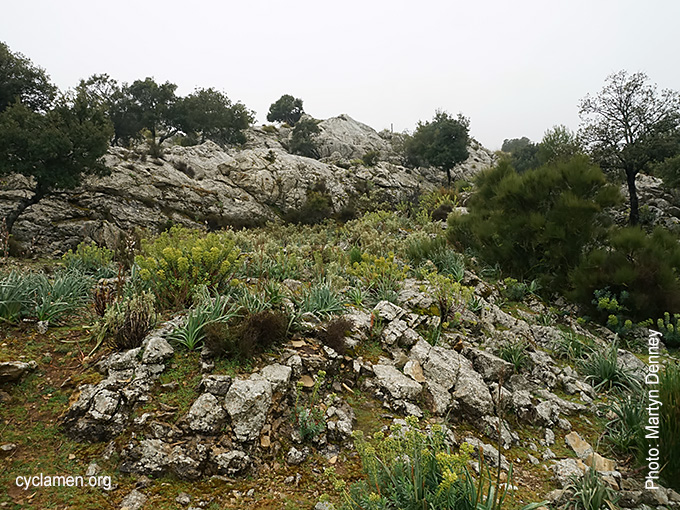The image captures a slightly gloomy, light gray sky over a rocky hill formation. Below the sky, the terrain features gray, cracked rocks with cut lines and jagged edges, some of which seem unstable. The hill is dotted with dark green trees, primarily fir types, along with shrubs, small ferns, and plants with yellow blossoms. There is also a patch of green grass at the base of the hill. A possible trail ascends diagonally up the rocky slope. In the bottom right-hand corner of the image, the photographer is credited as Martin Denny in white text, while the bottom left-hand corner mentions cyclamen.org, likely a website related to the image. The overall scene suggests a serene, natural setting, with a particular focus on both the rugged rock formations and the resilient plant life.